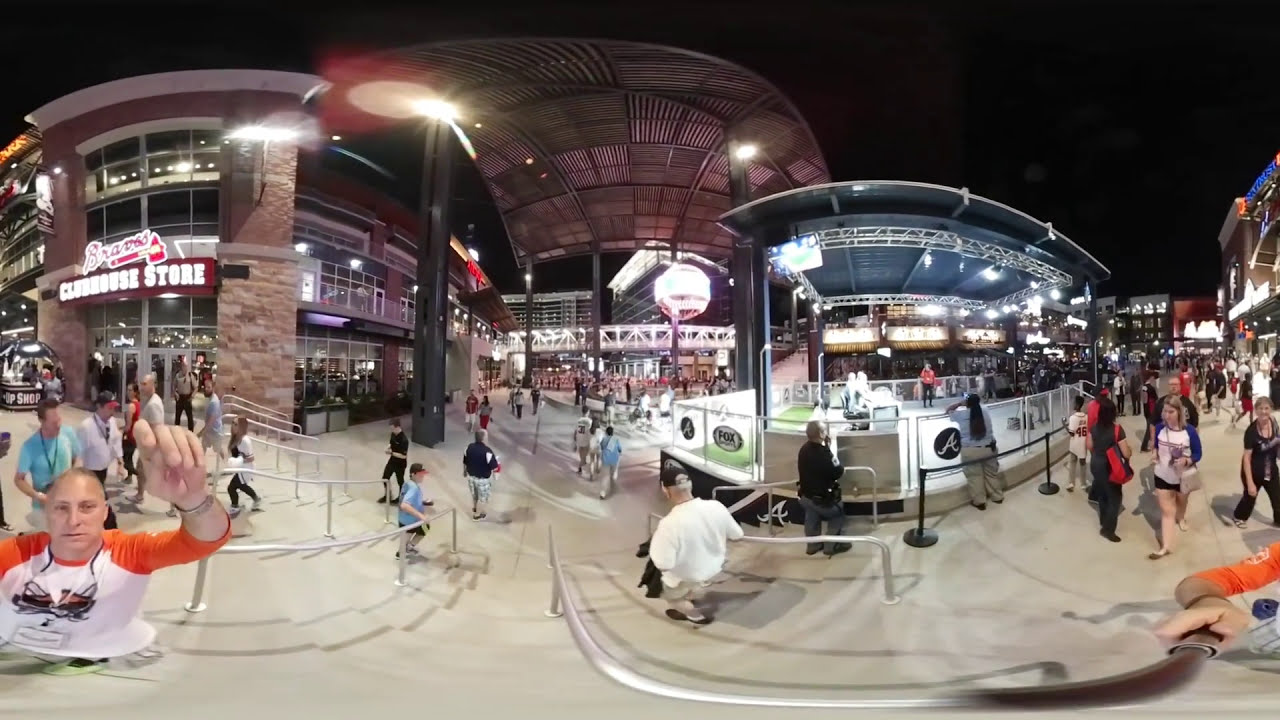The image captures a bustling nighttime scene outside the Atlanta Braves stadium, featuring a hard concrete floor and various scattered elements. Dominating the left side of the scene is the multi-story Braves Clubhouse Store, identifiable by its glass walls framed by brick pillars and illuminated signage. At the image's forefront, a man in an orange and white shirt with sunglasses, possibly the photographer, stands in the bottom left corner, facing the camera.

The environment is lively, with people milling around the area, funneled through entry points with metal railings that direct traffic. The central section of the image displays a mix of small stands and shops, hinting at the presence of vendors and restaurants. On the right-hand side, there's a small stage with individuals walking past. The atmosphere is dynamic and crowded, with no single focal point, illustrating the varied activities taking place. The color palette includes tan, orange, white, black, gray, silver, green, red, and blue, adding vibrancy to the scene. Additionally, there appears to be a section in the background where an Atlanta broadcaster or another enclosure is located, attracting onlookers. The overall setting suggests it is nighttime, with bright lights accentuating the architectural and human elements, encapsulating the vibrant ambiance of an evening at the ballpark.